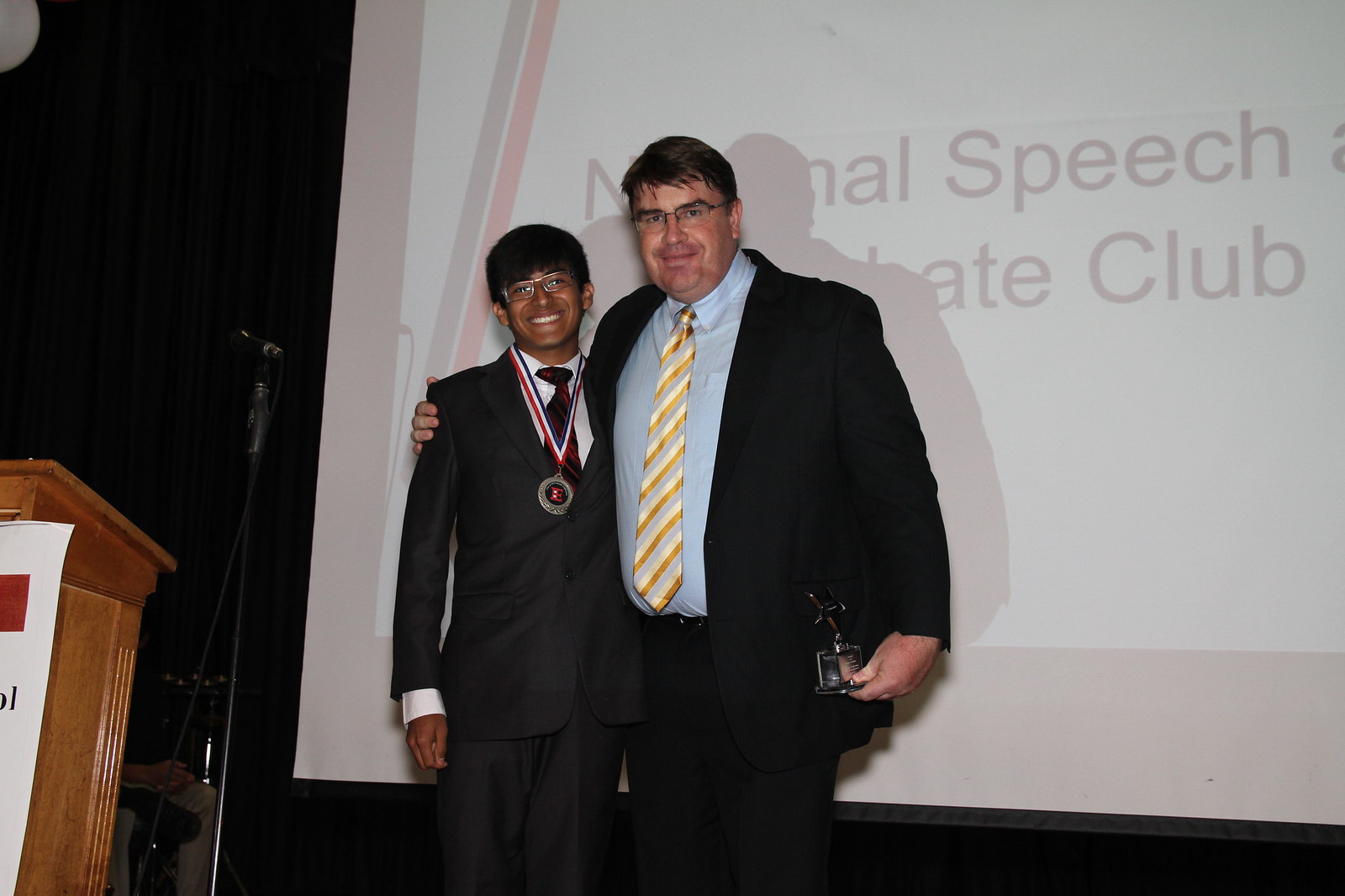This horizontal rectangular image captures a photograph of two males standing on a stage in front of a large white screen with partial text visible, displaying the words "speech" and "debate club." The person on the left is a young, short, and slight Indian teenager, approximately 14 years old, with short black hair and wire-rimmed glasses. He is dressed in a black suit with a white collared shirt and a black-and-red striped tie, smiling openly at the camera. Around his neck hangs a circular medal, indicating he has won a prize. The individual on the right is a large, heavyset white man in his 40s, donning a black suit, light blue shirt, and a yellow striped tie. He has short brown hair, wears glasses, and smiles with his mouth closed. His right arm is around the young man's shoulder, and he holds a small trophy in his left hand by his side. To the left of the frame, half of a wooden podium is visible, suggesting its use for speeches. Black stage curtains frame the scene, reinforcing the formal and celebratory atmosphere of a speech and debate club event.